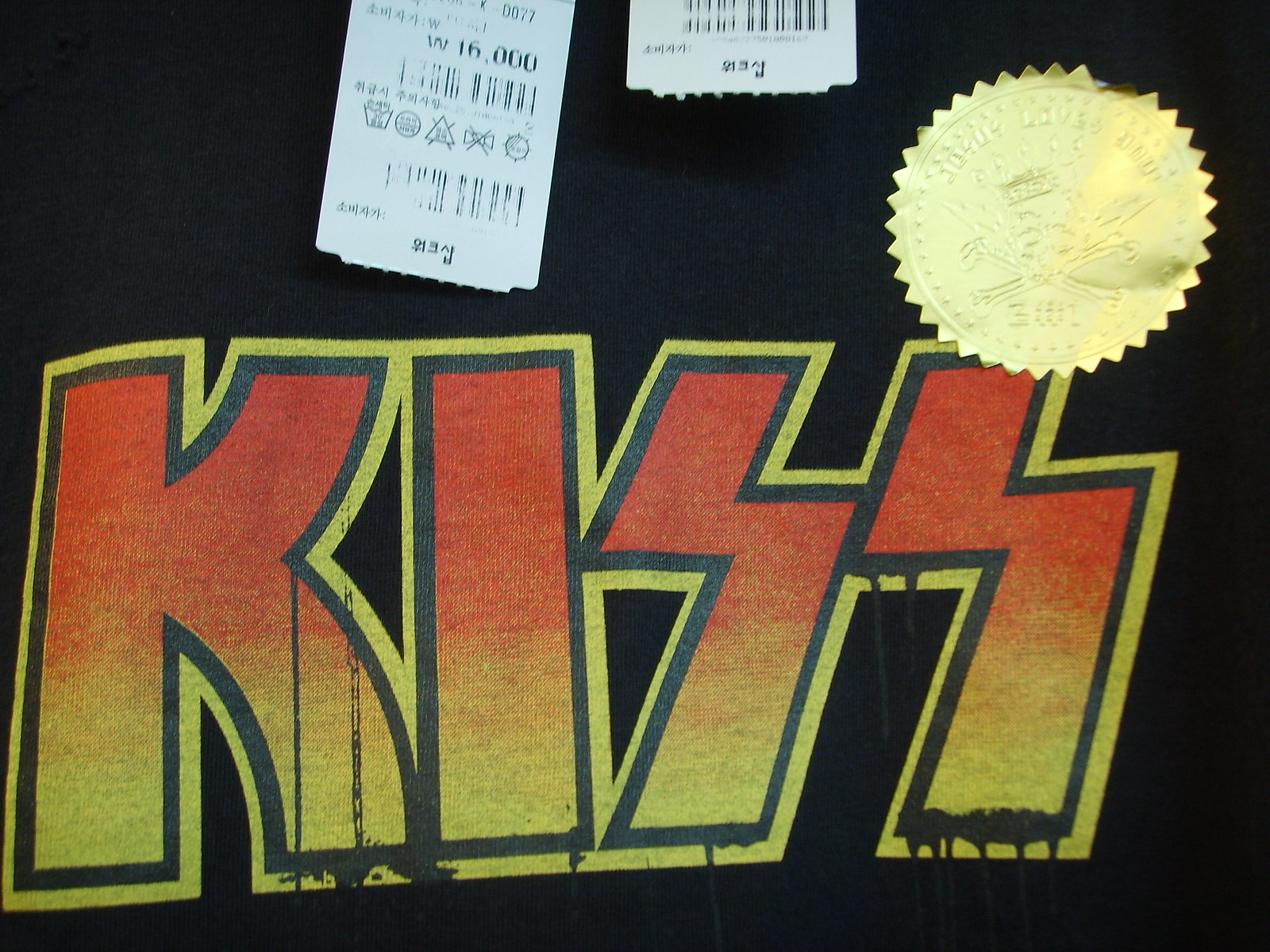This close-up photo features a black t-shirt adorned with a KISS logo, reminiscent of their album artwork. The logo, in bold red and yellow lettering with a black outline, spells out "KISS" with a notable melting effect at the bottom of the 'K' and 'S' letters as well as the corner of the first 'S.' At the upper right corner of the shirt, there is a glossy gold sticker, though its details are indistinct. The shirt also displays two white tags with black writing, positioned closely together, one to the left and the other in the middle. The tags indicate the price in Korean currency, suggesting the shirt is sold by a Korean retailer for 16,000 won. The design appears defective due to improperly pressed colors, causing the melting effect to extend onto the black fabric of the shirt.